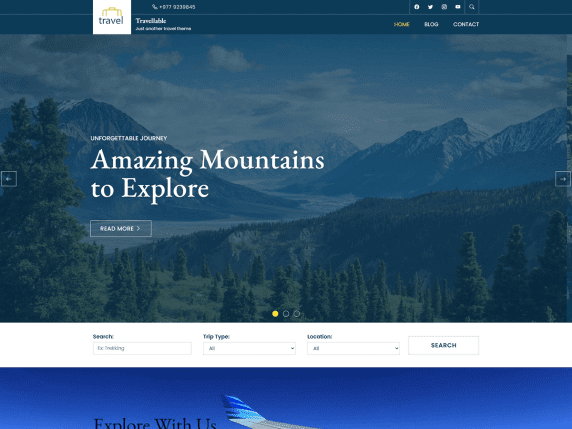A screen capture from a travel website is displayed, featuring an organized and visually appealing layout. At the top, a small box labeled "Travel" is accompanied by a suitcase icon, hinting at the website's purpose. Although the company's name is not clearly legible, the navigation bar prominently displays links to "Home," "Blog," and "Contact," along with a visible phone number for direct inquiries.

Dominating the main section of the page is a striking photograph of towering, snow-capped mountains, accompanied by a bold caption that reads, "Unforgettable Journey, Amazing Mountains to Explore." Directly beneath this inviting image is a "Read More" link, encouraging further exploration of mountain adventures.

Below the mountain image is another evocative photograph, this one capturing the tip of an airplane wing against a backdrop of an expansive sky. Partial text below this image reads "Explore with us," suggesting a call to action for potential travelers.

Between these two captivating photographs lies a functional search bar, flanked by dropdown menus for selecting "Trip Type" and "Location." A final "Search" button awaits to finalize the selection process, guiding users toward discovering their next adventure and booking their travel plans seamlessly.